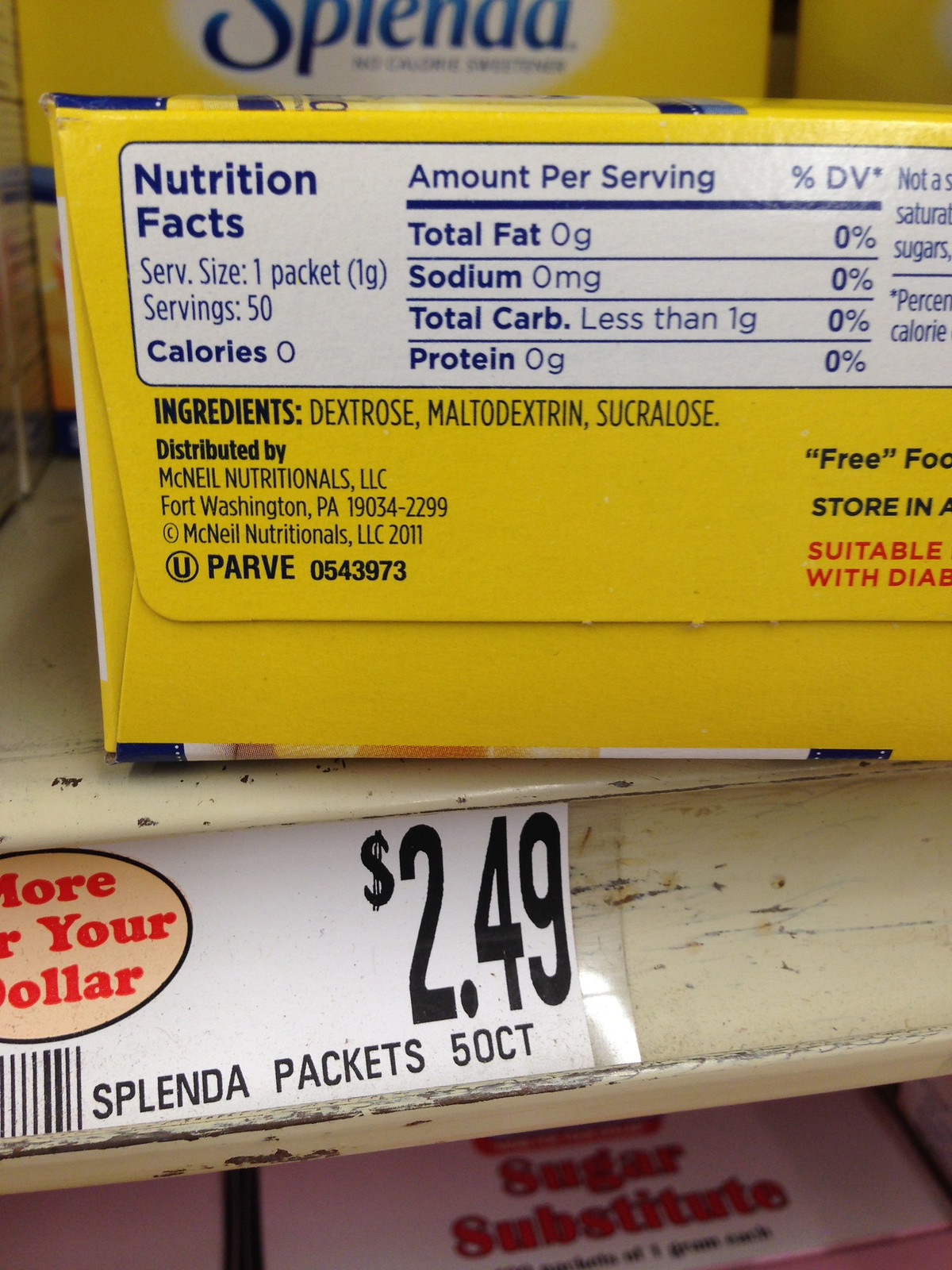A detailed photograph captured in an older grocery store prominently showcases the nutrition information and price tag of a Splenda packet. The price tag is affixed to the edge of a classic metal shelf, highlighting the message "More for Your Dollar." This label includes a UPC number, specifying "Splenda Packets, 50 Count" priced at $2.49.

In the main focus, the Splenda package is oriented on its side, drawing attention to its nutrition facts. Each serving size is a single packet, with a total of 50 servings per container. Notable nutrition details include zero calories, zero fat, zero sodium, less than one gram of carbohydrates, and zero protein. The ingredient list mentions dextrose, maltodextrin, and sucralose, with distribution by McNeil Nutritionals, LLC.

Additional package information mentions "free food" and instructs storage and usage, though these directions are partially obscured.